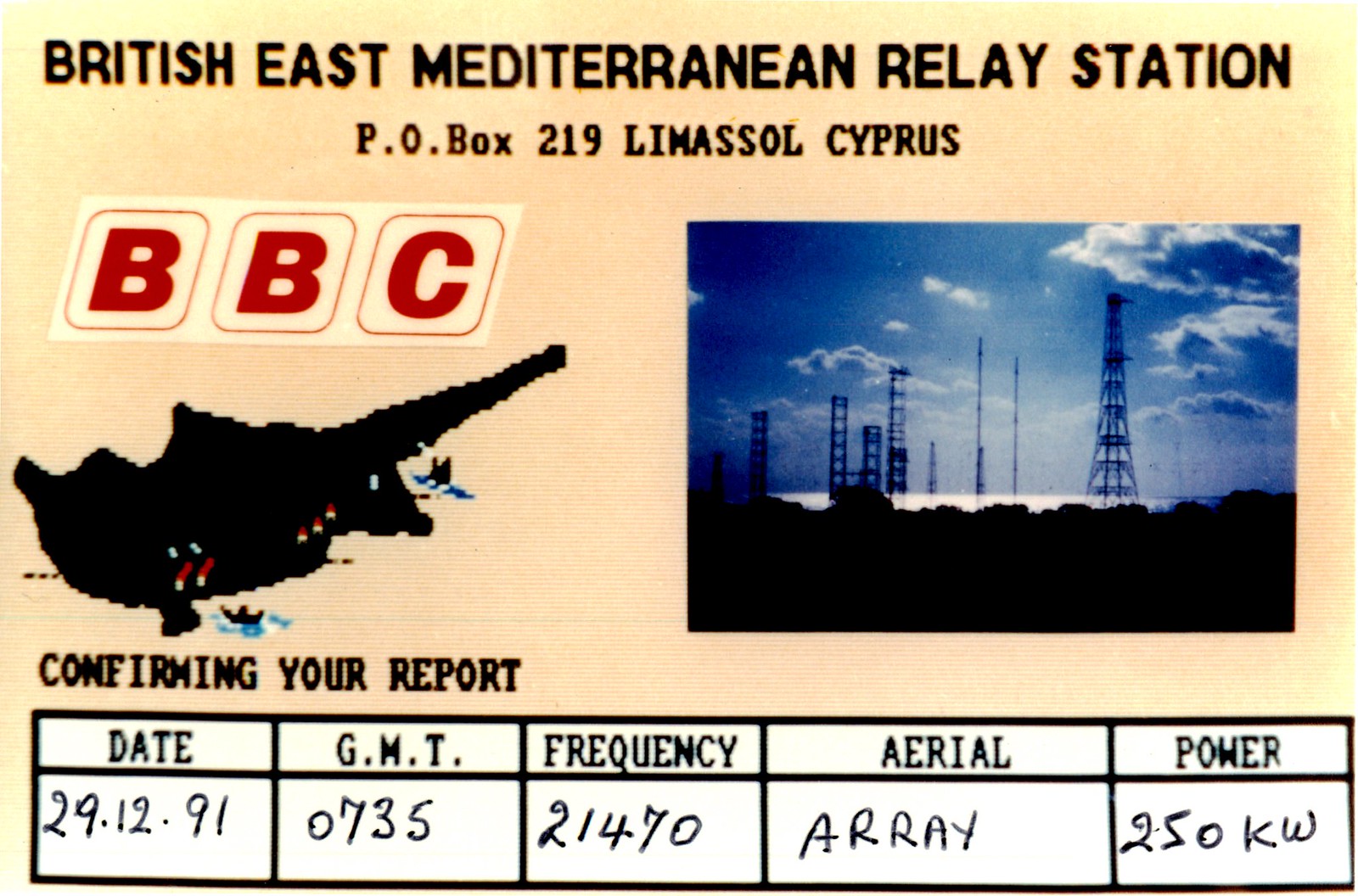The image is a scanned postcard from the 1990s with a light blue background that has a fine line texture. At the top, it reads "British East Mediterranean Relay Station" followed by the address "Fuel Box 219, Limassol, Cyprus." The BBC logo, presented in red and white, is prominently featured. Below this, there is a complex image that includes a dark shape with red symbols, possibly depicting a location or country, next to a photograph of relay or radio stations set against a blue sky with darkened clouds. The ground in the photo appears very dark, almost black. Additionally, the postcard includes detailed information: "Confirming your report" is stated at the bottom, alongside the date "12-29-91, GMT (Greenwich Mean Time) 735," the frequency "21470," and mentions of an "aerial array" with a power of "250 kilowatts." The overall card is modestly colorful with a predominantly beige color and other colors sprinkled throughout.